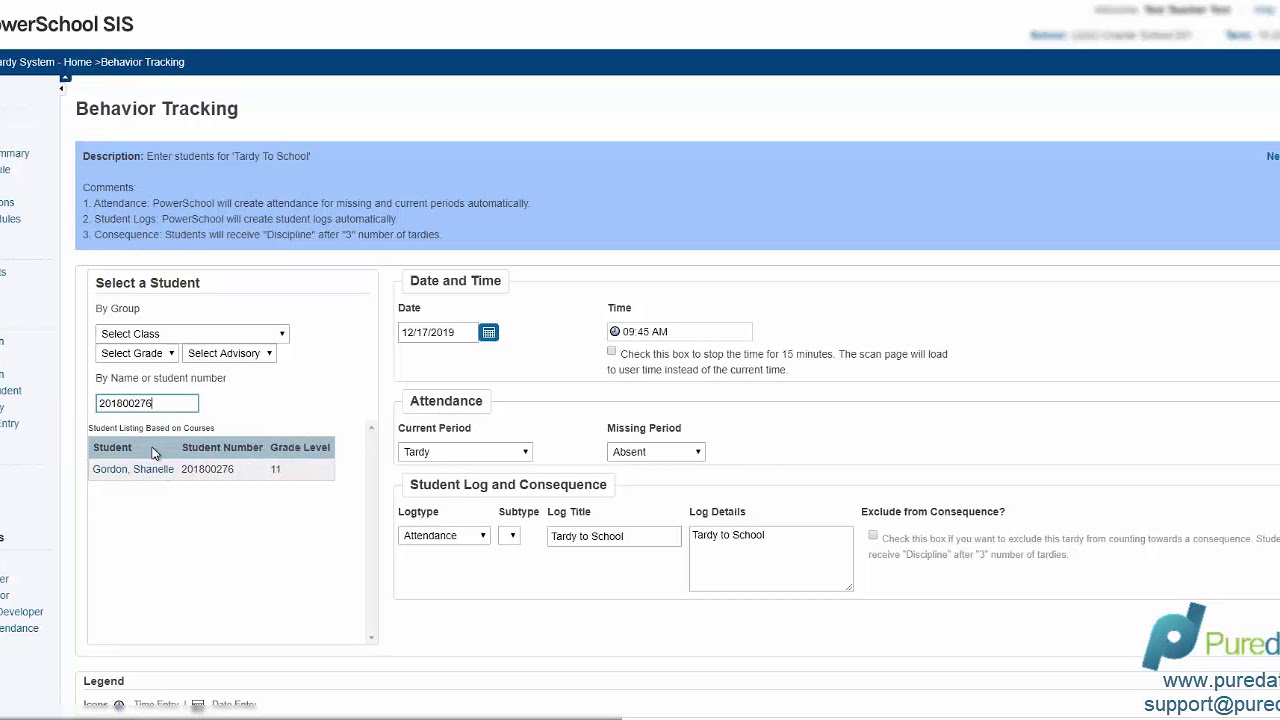The image displays a user interface on a white background for a school behavior tracking system. The top section contains the text "POWER" (missing the "P"), and underneath, "SIS," referring to a School Information System. The main section includes various interactive elements with detailed labels and fields.

There is a dropdown menu or selection box labeled "Select a Student by Group" and another rectangular selection for "Select Class." Below these, there are two more rectangles marked "Select Grade" and "Select," with an additional field for "BASRI" selection either by name or student number. A dedicated box is available for number input, with a cursor visible right after the last number entered.

A gray box with a blue header is prominently displayed below these choices. The header includes the columns "Student," "Student Number," "Grade Level," along with a pointer visible on the blue header. While "Student Name" and "Student Number" fields contain obscured text that is too small to read, the "Grade Level" field shows the number 11.

To the right-hand side, there are fields showing the "Date" (either 12/17/2019 or 11/17/2019) and "Time" as 9:46 AM. There are specified attendance statuses listed: "Current Period," "Tardy," "Missing Period," "Absent," and sections for "Student Log" and "Consequence." The area designated "Log Details" includes an entry of "Tardy to school." The section ends with an option labeled "Exclude from Consequence," which has a checked box with a question mark next to it.

Overall, the screen provides a comprehensive view of a student information system, focusing on attendance and behavior tracking, with multiple interactive elements for user input and detailed fields for student data.